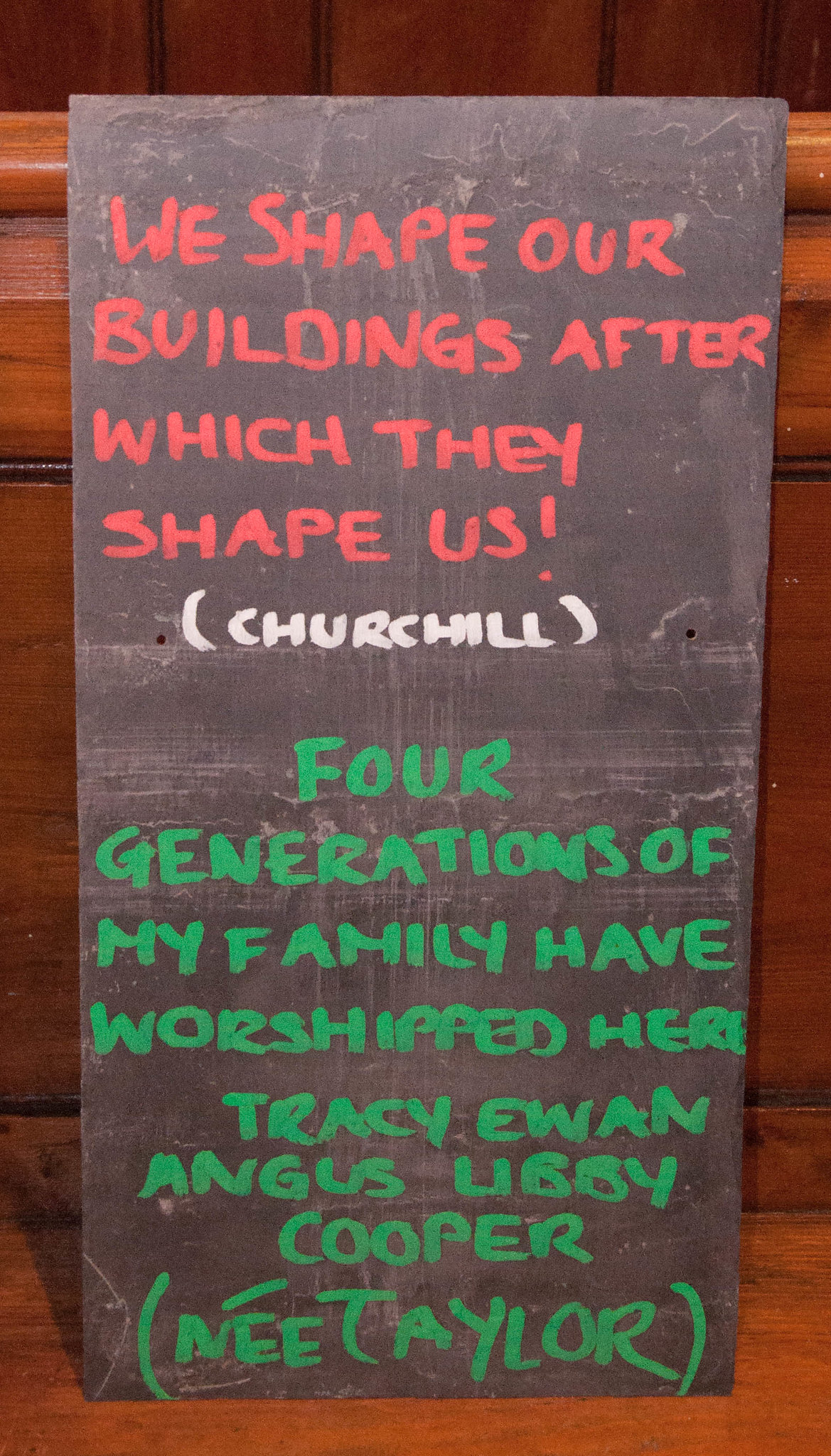The image depicts a vertically oriented black chalkboard-like sign resting against a wooden church bench or similar structure. The sign features a quotation in various colored writings. At the top, in red letters, it reads, "We shape our buildings, after which they shape us!" attributed to "Churchill" written in white letters just below. The lower portion of the sign, in green letters, says, "Four generations of my family have worshipped here: Tracy, Ewan, Angus, Libby, Cooper," followed by "Nee Taylor" in parentheses. The background is wooden, emphasizing the sign's placement in a rustic or traditional setting.